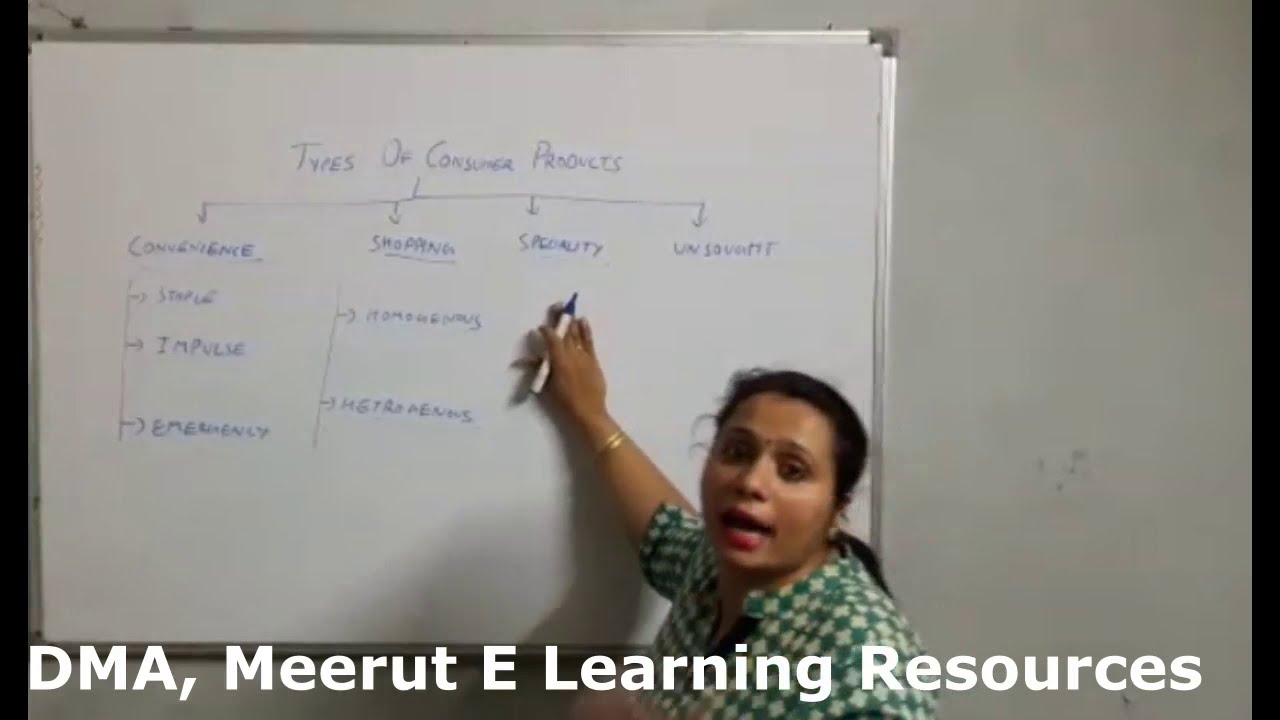The image captures a woman, likely a teacher, standing in front of a whiteboard, engaging with her audience. She faces the camera with her right hand raised to point at the whiteboard, holding a marker. The woman has a green and white checkered shirt, red lipstick, and her black hair pulled back in a ponytail. A gold bracelet adorns her wrist. The whiteboard, featuring a silver border, displays a chart titled "Types of Consumer Products" written in blue marker. The chart includes categories like "Convenience," "Shopping," "Security," and another fuzzy term, with subcategories such as "Impulse" and "Emergency" under the second column. The background of the image includes a white wall, and a thin black border frames the left and right edges of the picture. At the bottom of the photo, white lettering reads "DMA, Merit eLearning Resources."